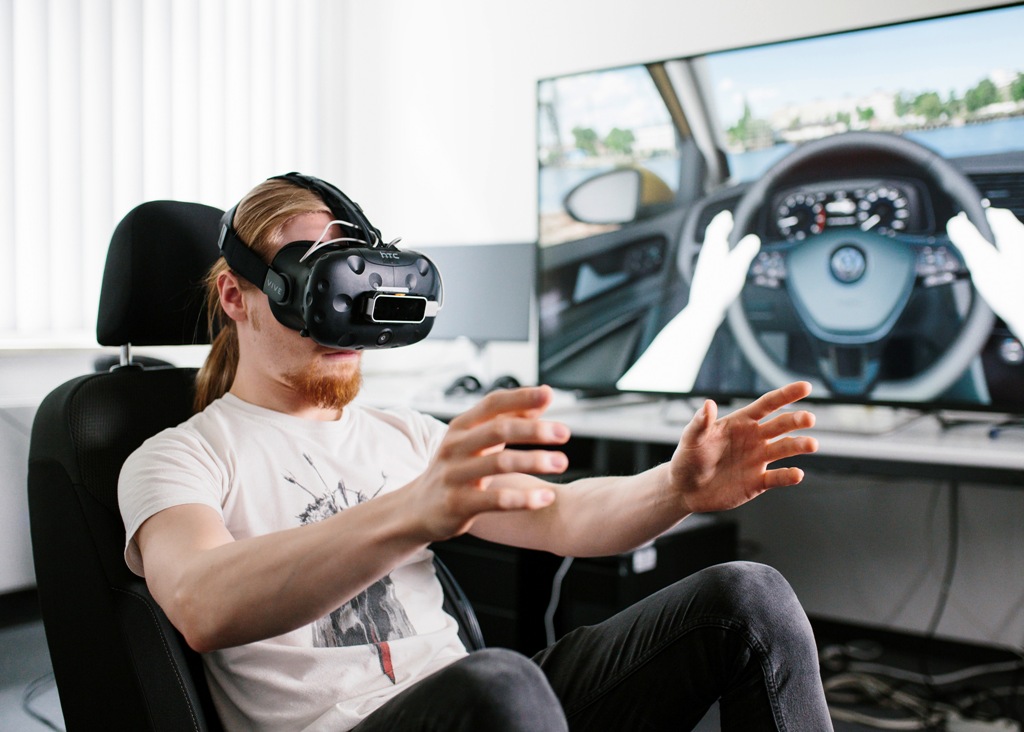In the indoor image, a man seated in a black chair, dressed in a white short-sleeved t-shirt and black skinny jeans, is immersed in a virtual reality experience. He wears black VR goggles that cover his eyes and extend over his head, with his long orange hair and orange goatee visibly contrasting against the white walls in the background. His arms are extended in front of him, as if gripping an invisible steering wheel, mimicking the sensation of driving a car. This simulated activity is confirmed by the large monitor to the right of the image, which displays a driving scene with a steering wheel and a car dashboard. Underneath the monitor, a keyboard rests on a desk, entangled with numerous wires. Behind the man, vertical blinds allow light to filter into the room, further illuminating the scene.